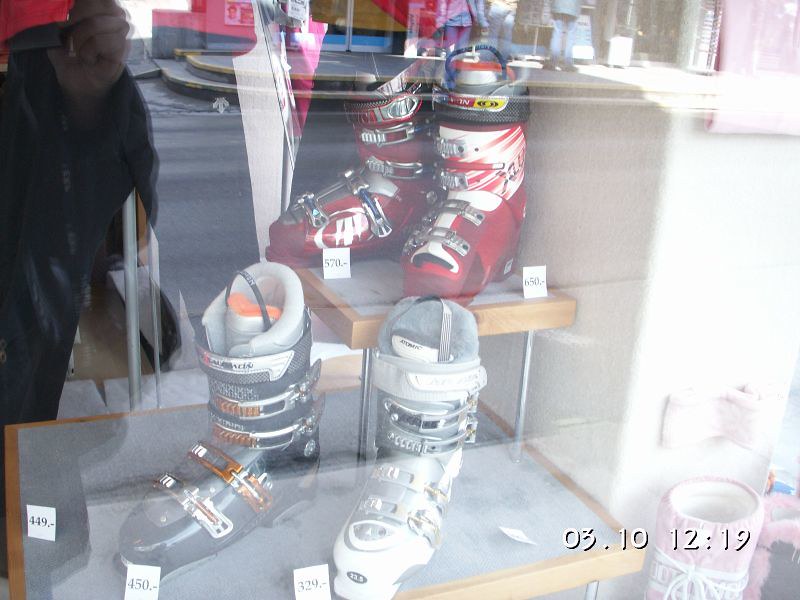This image captures a scene from the perspective of someone standing outside a store, looking through a glass display window. The reflection on the glass partially shows the street outside, including another shop across the road, and the photographer, who is wearing a black jacket and holding something in their hand. 

In the bottom right corner of the glass, white text reads "03.10 12;19," likely indicating the date and time the photo was taken. The display inside the window features a collection of boots on two shelves. The top shelf hosts a pair of deep red boots adorned with silver buckles and white price tags. The bottom shelf showcases a black boot with metallic bands on the left and a chunky grey boot with silver clasps on the right. Additionally, several prices are listed at the bottom of the display: 6.50, 7.50, 4.49, 4.50, and 3.29. The overall appearance of the boots suggests that they could be skiing boots or some type of sporty, medical footwear.